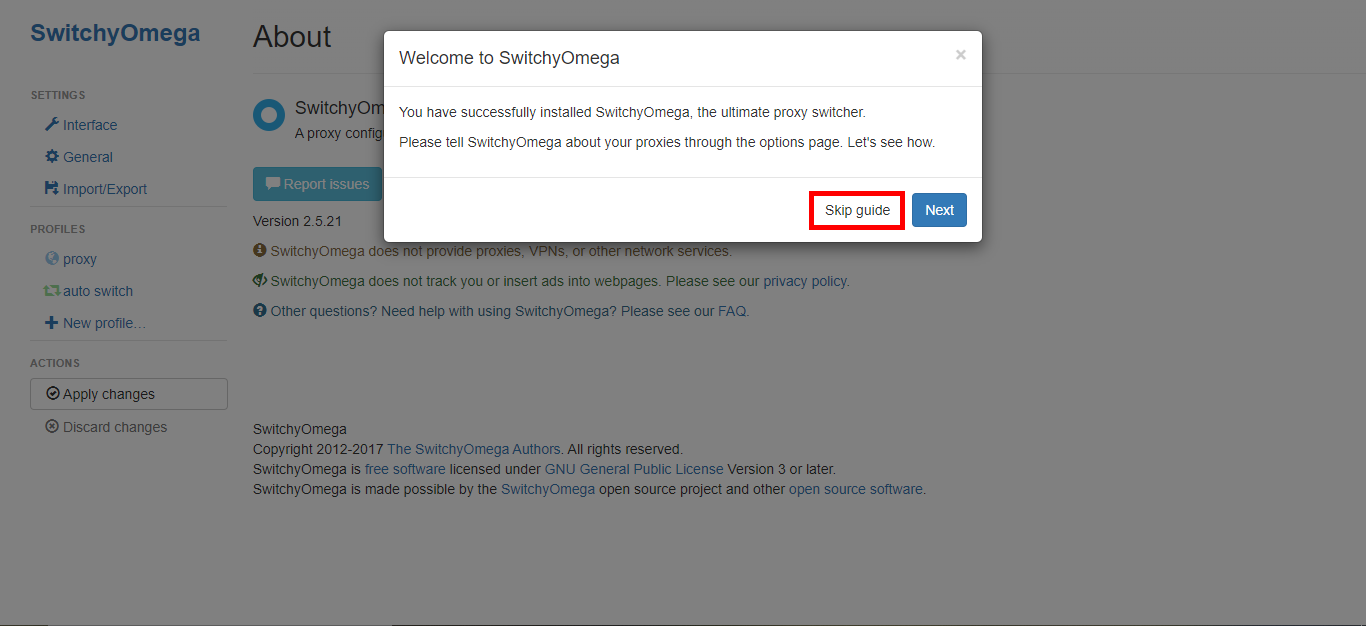The image is a screenshot from the SwitchyOmega application. Dominating the screen is a prominent pop-up window with the message: "Welcome to SwitchyOmega. You have successfully installed SwitchyOmega, the ultimate proxy switcher. Please tell SwitchyOmega about your proxies through the options page. Let's see how," accompanied by a circled option for "Skip Guide" highlighted in a red rectangle and a blue "Next" button.

The main interface in the background is displayed on a medium to light blue backdrop. At the upper left corner, "SwitchyOmega" is prominently titled in blue. A side menu on the left features several sections under "Settings," including "Interface," "General," and "Import/Export." Under "Profiles," there are "Proxy," "Auto Switch," and an option to create a new profile indicated by a plus sign. The section also contains action buttons labeled "Apply Changes" and "Discard Changes."

Partially visible beneath the pop-up window is a section labeled "About," displaying the SwitchyOmega icon and the beginning of the phrase "a proxy config," with other details obscured. A blue button for reporting issues is also visible.

Towards the lower portion of the screen, the version number "2.5.21" is indicated alongside an informational note: "SwitchyOmega does not provide proxies, VPNs, or other network services." Additionally, a green icon emphasizes that "SwitchyOmega does not track you or insert ads into web pages," with a clickable link to the privacy policy. A question mark icon next to it offers further assistance and guides users to the FAQ section via another blue link.

At the bottom of the screenshot, a copyright notice reads: "SwitchyOmega © 2012 to 2017 SwitchyOmega authors. All rights reserved. SwitchyOmega is free software licensed under GNU General Public License version 3 or later. SwitchyOmega is made possible by the SwitchyOmega open source project and other open source software."